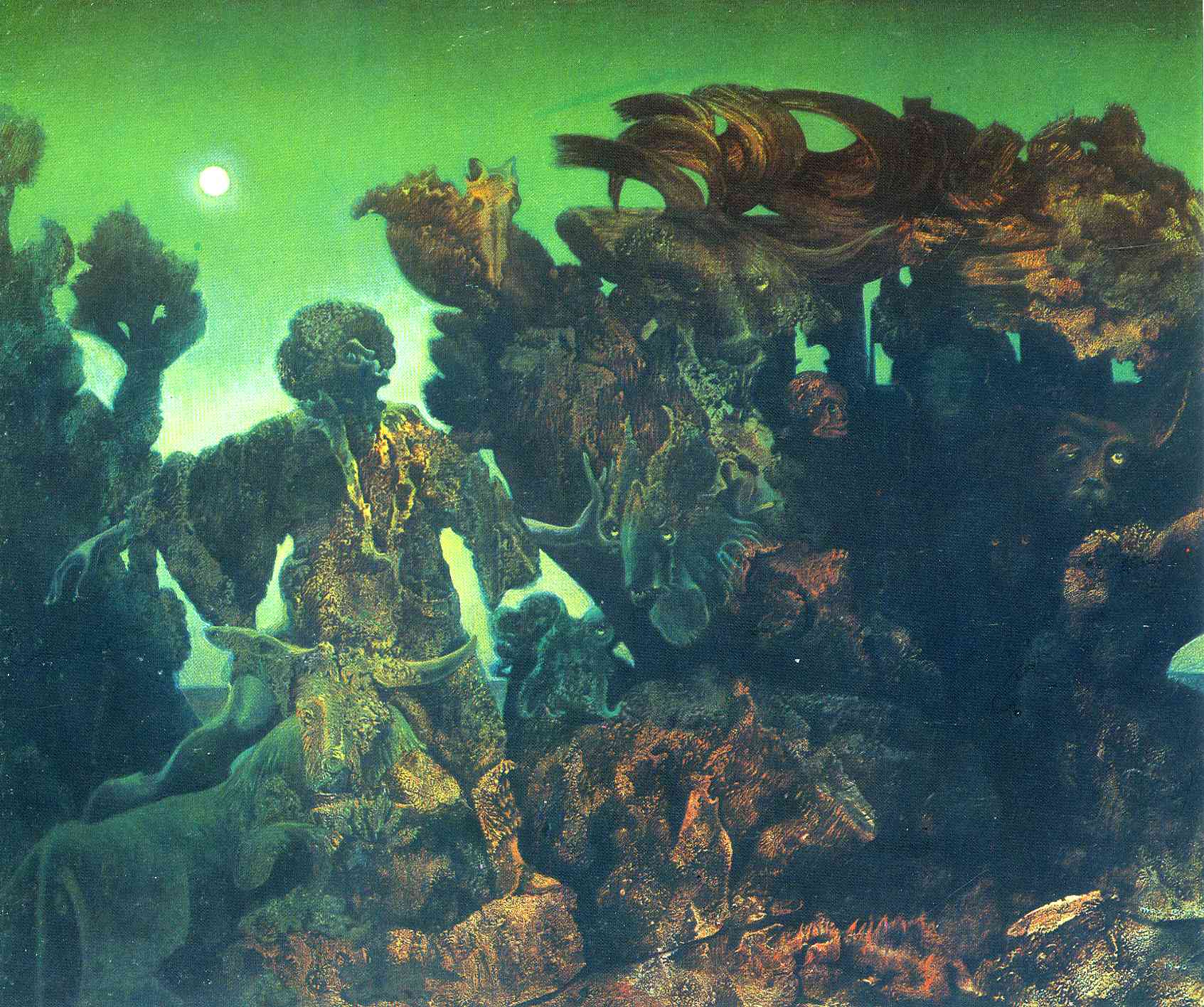This surreal artwork is an intricate, ethereal painting that captures what initially seems to be an underwater coral scene. Upon closer inspection, the scene is revealed to be a fantastical, alien landscape blending various elements. The background is predominantly parrot green, evocative of an unconventional sky, with a small white circle in the upper left corner representing a moon or sun. The foreground features an array of rocky formations imbued with fantastical, dark-hued designs.

In the center of the painting stands a prominent humanoid figure, draped in flowing robes and adorned with a puffed, elaborate hairstyle. This figure appears to be observing a large structure to the right, composed of a whimsical mixture of animal and human elements—a motif recurring throughout the artwork. On the bottom left, a distinctly horned cow or ox figure embellishes the rocky terrain, while to its right is an octopus and a fish design. In the background, various animal heads, such as a bear with leaves sprouting from it and possibly coyotes, subtly emerge from the stone. Additional mysterious faces and eyes, perhaps feline, peer out from cavern-like recesses, enhancing the painting’s surreal and composite nature.

Overall, the piece uses a palette of browns, blues, greens, golds, and occasional touches of red to build an elaborate, surreal tapestry. The detail and seamless blending of elements create a captivating visual experience that reveals more the longer one looks, transforming a simple coral wreath scene into a complex, otherworldly vista.